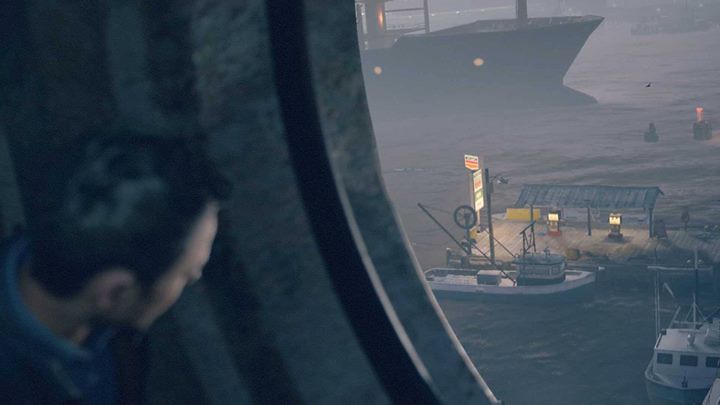"A contemplative Caucasian man, approximately 30 years old with short brown hair, gazes out of an industrial-style porthole on the left side of the image. His side profile is sharply detailed against the misty, moody backdrop of a harbor at either dusk or dawn. The harbor scene reveals a cluster of small working boats docked along a weathered pier. In the foreground, a tugboat rests beside a dock, which also hosts a fishing boat positioned at an angle. Prominently visible are illuminated gas pumps beneath a simple shelter, accompanied by a glowing sign advertising the fuel. Further in the distance, the bow of a larger ship looms, partially shrouded in the haze, amidst a scattering of additional vessels. The calm seawater reflects the muted ambiance, enhancing the serene yet industrious atmosphere of the harbor."